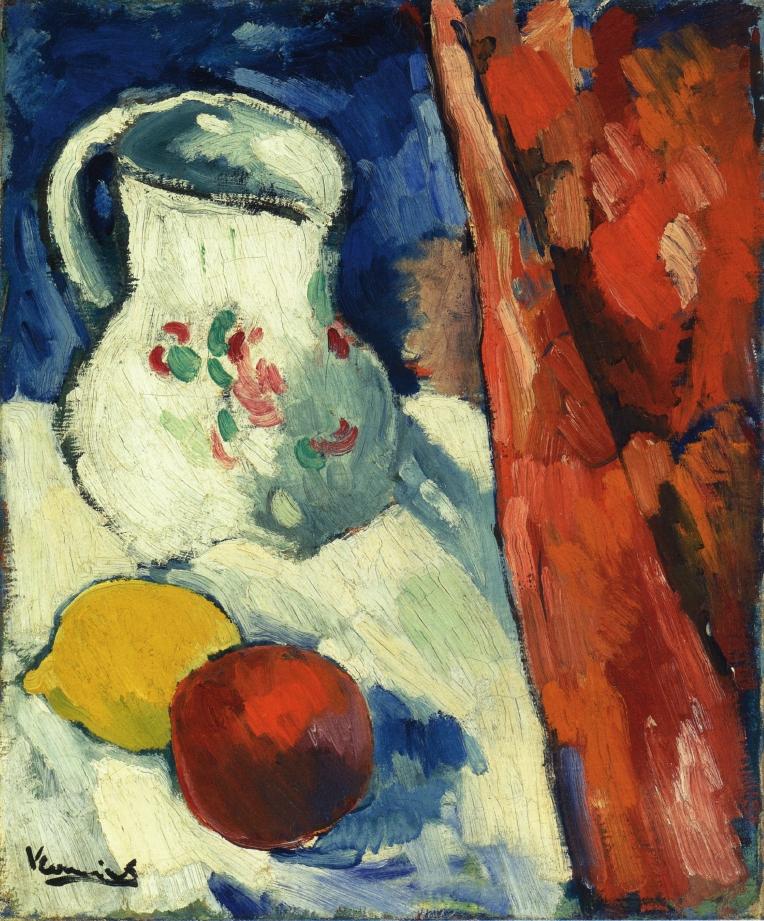The painting, in an Impressionist style attributed to Vermeer, showcases a still life scene centered around a pristine white tabletop. Atop the table sits a white pitcher adorned with floral motifs and outlined in black, casting a bluish shadow. Beside the pitcher, two pieces of fruit are carefully placed: a bright yellow lemon to the left and a reddish apple or peach to the right. The background is composed of deep blue hues that transition from midnight blue to lighter shades with white highlights. To the right, a wooden oar diagonally spans from the top to the bottom of the painting, while in the background, rich red and dark copper tones blend seamlessly with blue and umber accents. The foreground features a white tablecloth tinged with green and yellow hues. The bottom left corner of the painting bears an indistinct signature.